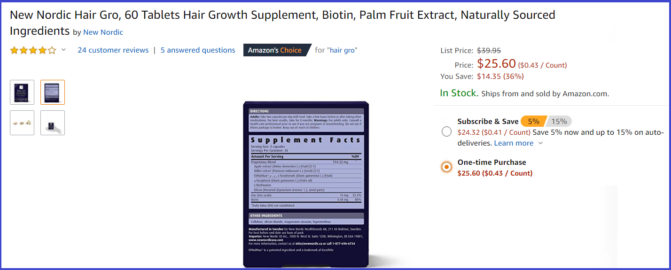Screenshot of an Amazon.com product selection page bordered by a blue line. The top left features the product name in black font: "New Nordic Hair Grow, 60 Tablets Hair Growth Supplement, Biotin, Palm Fruit Extract, Naturally Sourced Ingredients." The brand "New Nordic" is indicated below. 

Customer feedback is summarized with a rating of 4 out of 5 stars from 24 customer reviews and 5 answered questions. There is a badge combination with a black rectangle reading "Amazon" in white font, followed by "Choice" in yellow font, and "for 'Hair Grow'" in blue font.

The pricing details include a crossed-out list price of $59.95, with a current price displayed in red font as $25.60 (equating to 45 cents per tablet). The discount saves customers $34.35, a 56% reduction. The product status indicates "In Stock" with shipping details initially obscured.